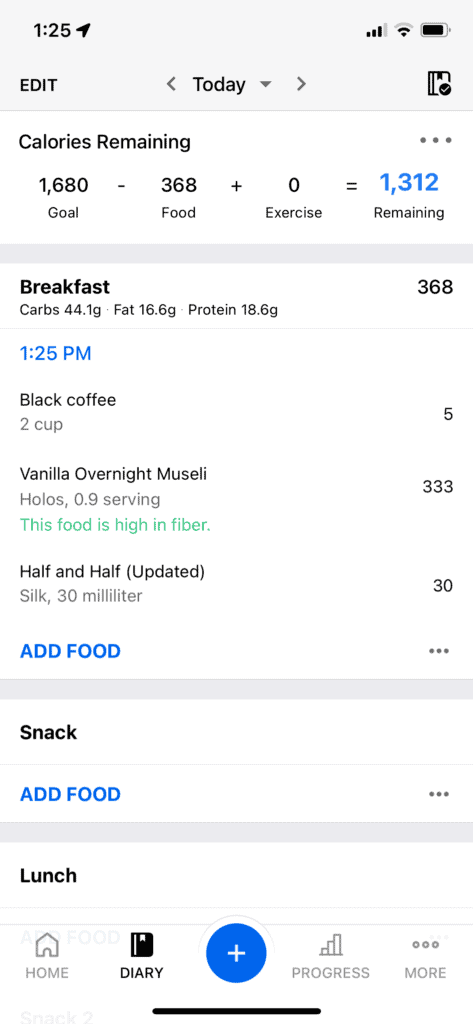This is a detailed screenshot of a mobile diet-tracking app, likely viewed on an iPhone given the interface design. The app features a minimalist and simplistic aesthetic, predominantly using white as its main color. At the top, the screen displays "Today," indicating that this is the food diary for the current day.

Below this heading, the app provides a summary of the user's caloric intake: a goal of 1680 calories minus 368 calories consumed, plus calories burned from exercise (which currently stands at zero). This results in 1312 calories remaining for the day, suggesting that the user still has a significant portion of their daily allowance left.

The user's food diary shows entries for breakfast, including "Coffee," "Vanilla Overnight Muesli," and "Half and Half." While breakfast has been logged, entries for other meals such as snacks and lunch have yet to be added.

A navigation bar is located at the bottom of the screen with five icons: "Home" on the far left, "Diary" (currently selected), a central blue plus sign for adding new entries, "Progress" to track goals and milestones, and "More" for additional options. The organized layout and clean design make it easy for users to track and manage their dietary intake throughout the day.